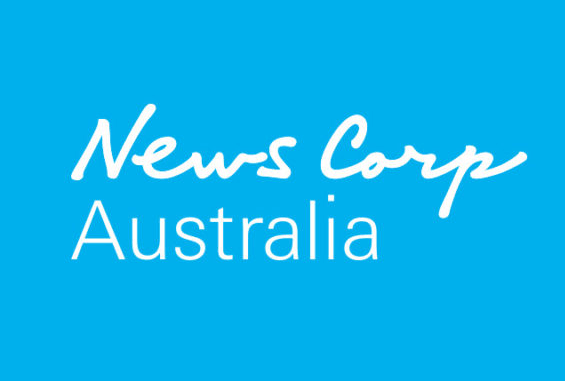The image features a bright sky blue rectangular background that is longer horizontally than it is vertically. Centered prominently in the rectangle is the text "News Corp Australia." The "News Corp" portion is written in a stylized, cursive font with thick line weight, conveying a sense of elegance and formality. Below this, the word "Australia" appears in a more conventional, computer-typical typeface, providing a straightforward and easily readable contrast to the cursive script above.

The text is centrally aligned within the rectangle, with generous margins on the top and bottom compared to narrower margins on the sides, particularly with a slightly smaller margin on the right than on the left. The visual design is clean and simple, with a high contrast between the bright blue background and the white text, making the words stand out clearly.

There are no additional elements or embellishments; the focus remains solely on the "News Corp Australia" text. Notably, in the word "News," the cursive "W" does not connect fully to the "S," adding a unique touch to the otherwise flowing script. The overall design is modern and professional, emphasizing the branding of "News Corp Australia."